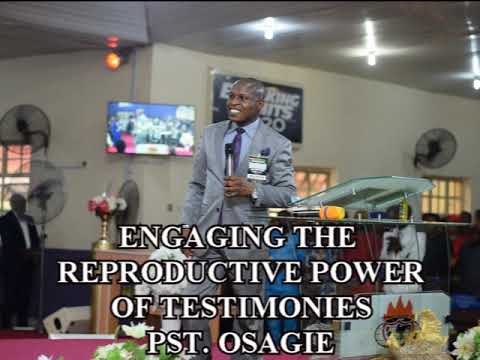The image shows a man of African-American descent, possibly a preacher, inside a brightly-lit church. The photo, cropped to a square shape, centers on him as he stands smiling with a microphone in his left hand. He is bald and wears a grey suit paired with a light blue button-down shirt and a purple tie. The background reveals a white wall with fans mounted on it, a TV screen in the corner likely displaying a choir, and another man in a black suit on the left. The bottom of the image features flowers and prominently displays white block lettering that reads, "Engaging the Reproductive Power of Testimonies, PST, Osagie." The room's high ceilings and bright lighting add to the vibrant atmosphere, focused on the preacher as he engages with his audience.